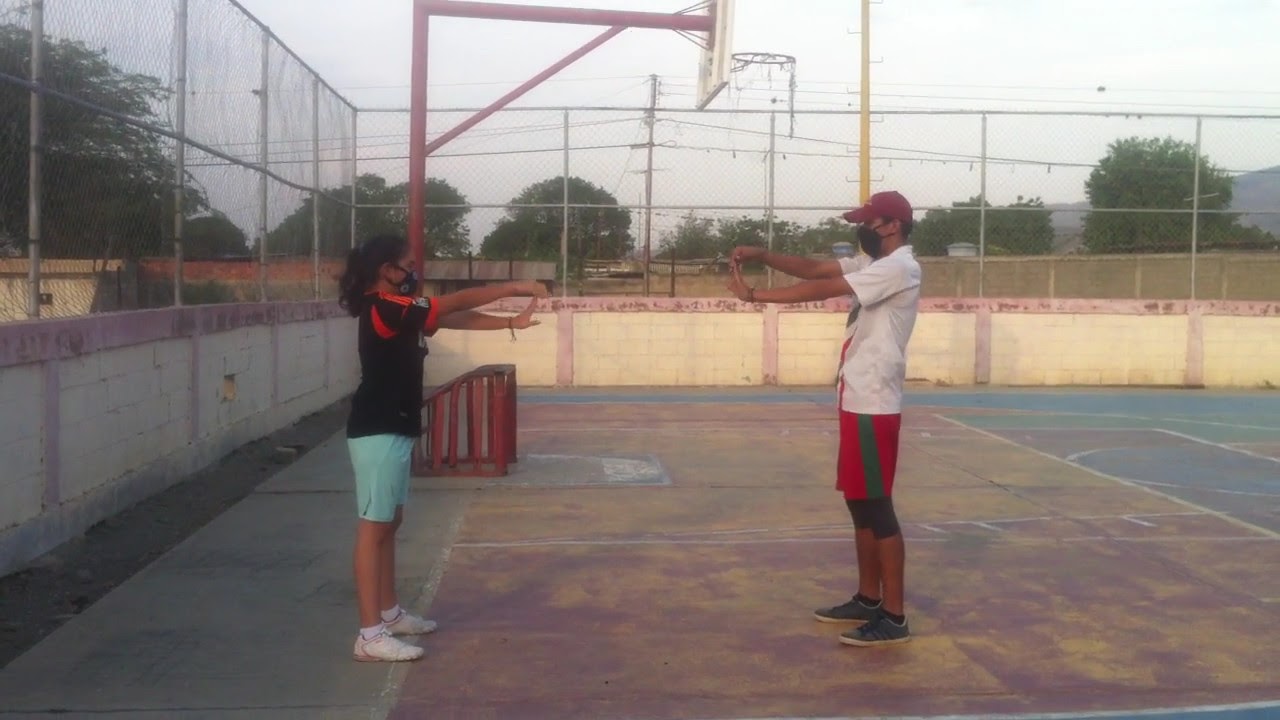In this outdoor daytime photograph, two individuals are seen on a fenced-in basketball court, apparently engaged in stretching exercises. The court features a clear view of the basketball hoop and the surrounding netting. The background reveals a scenic array of trees, distant hills, buildings, and electric poles under an overcast sky, suggesting a Southeast Asian locale.

The male on the right, possibly a coach, is outfitted in a white t-shirt, red and green shorts with black knee-length shorts underneath, grey sneakers, and black socks. He is also wearing a maroon baseball cap and a black face mask. His left hand is stretched out, with his right hand pulling back the fingers of his left. Opposite him stands a female, likely an athlete or perhaps his daughter, given her slender build and ponytailed black hair. She dons a black t-shirt with red accents on the sleeves, turquoise blue shorts, white sneakers, and a black face mask. She mirrors the man's stance, stretching her left hand with her right.

Both individuals, showcasing dark brown skin, are positioned facing each other, contributing to a scene enveloped in the shared activity of stretching amidst a vividly colored court and a picturesque backdrop.